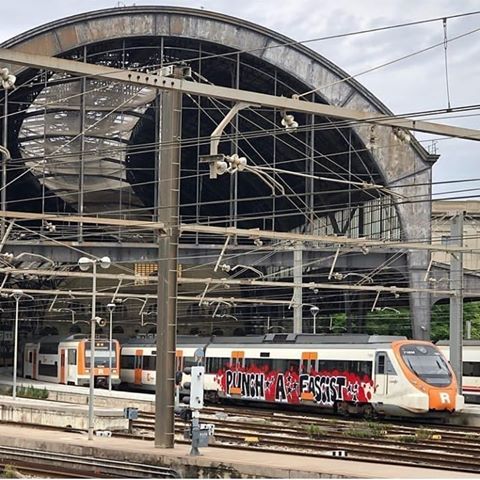This vibrant color photograph captures an outdoor daytime scene featuring two monorail trains. Dominating the frame, the primary monorail travels rightward and boasts a sleek white exterior accented with orange trim. An "R" is prominently displayed beneath its main window. Distinctively, the monorail's side is heavily adorned with graffiti; a bold, black, capitalized message reads "PUNCH A FASCIST," highlighted by a white outline amidst red spray paint.

In the background, a second, more distant monorail echoes the primary one's path. Towering behind both trains is a large, arched structure, its height accentuated by the intricate web of crisscrossing wires. This architectural marvel stands tall and open, creating a dynamic contrast with the natural greenery that peeks from behind the primary monorail. The lush vegetation adds a touch of serenity to this urban tableau.